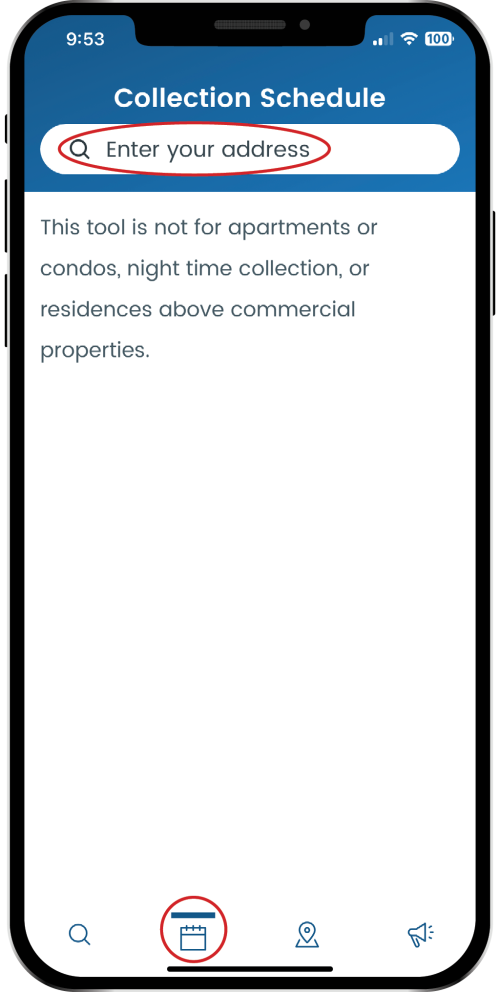Screenshot of a prototype iPhone interface showing a "Collection Schedule" page. At the top, within a blue banner, there is a rounded rectangular field labeled "Enter Your Address," highlighted by a red oval. Below the blue banner, a notice states: "Tools are not for apartments, condos, nighttime collection, or residences above commercial property." Towards the bottom of the screen, a calendar icon is encircled for emphasis. Adjacent to this icon are a magnifying glass, a location pin, and a sound icon. Additional details include indicators showing the battery fully charged to 100%, Wi-Fi enabled, signal strength with two bars, and the current time displayed as 9:53.